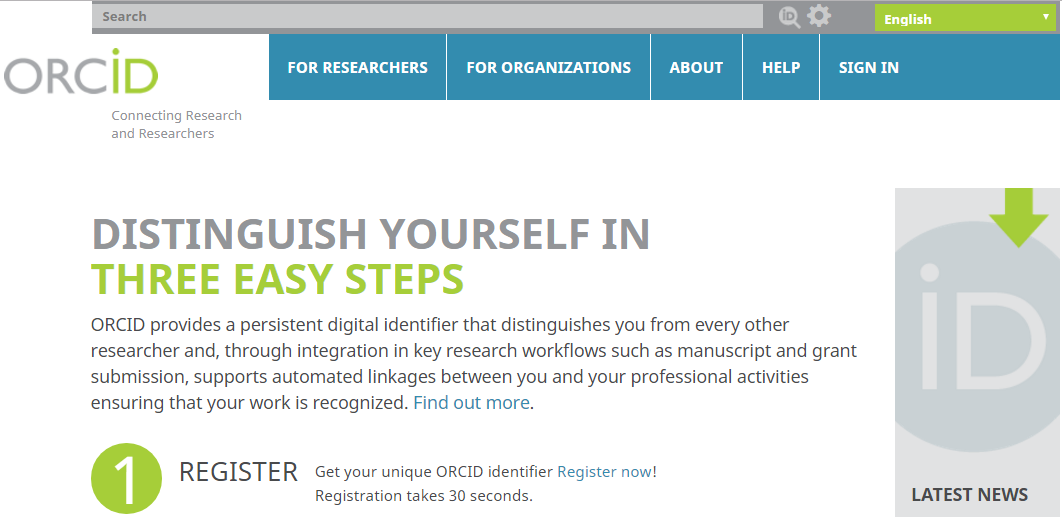Screenshot Description: 

The screenshot appears to be from the ORCID website, a platform designed to connect researchers and developers. The header of the page features a search bar and several navigational tabs labeled: Researchers, Organizations, About, Help, and Sign In.

The main content centers around the headline, "Distinguish Yourself in Three Easy Steps." It introduces ORCID as a service that provides a persistent digital identifier, which uniquely distinguishes each researcher. This identifier is integrated into key research workflows, such as manuscript and grant submissions, to support automated linkage between researchers and their professional activities, ensuring their work is properly recognized. 

Beneath this introduction, there's a hyperlink inviting users to "Find out more." Below it, a large numeral "1" marks the first step of the process. The step is titled "Register," prompting users to obtain their unique ORCID identifier. Another hyperlink reads "Register now," emphasizing that the registration process takes only 30 seconds. The right side of the page features an icon labeled "ID Latest News."

The overall layout is clean and organized, guiding users through the process of registering for an ORCID identifier with clear instructions and easy-to-follow steps.